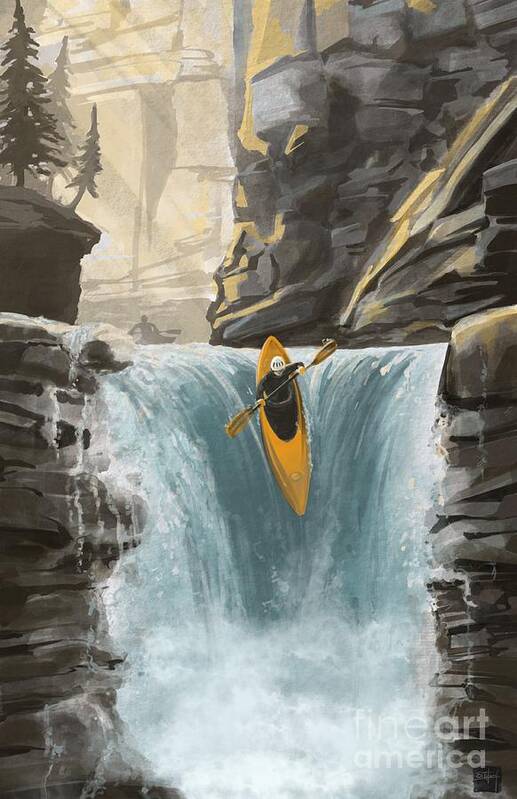The painting captures an exhilarating outdoor scene where a kayaker navigates a steep, blue-water waterfall set within a rugged, mountainous landscape. The central focus is a person in a bright yellow, one-man kayak descending the waterfall, with foamy water gushing at the bottom. The kayaker, dressed in a dark wetsuit and white helmet, grips a yellow oar in both hands. Above them, imposing rocky cliffs and mountainsides frame the cascade, with pine trees on the left side, where rays of sunlight filter through. In the background, the shadowy outline of another kayaker approaches the drop-off. In the lower right-hand corner, the watermark "Fine Art America" is subtly inscribed in block font.